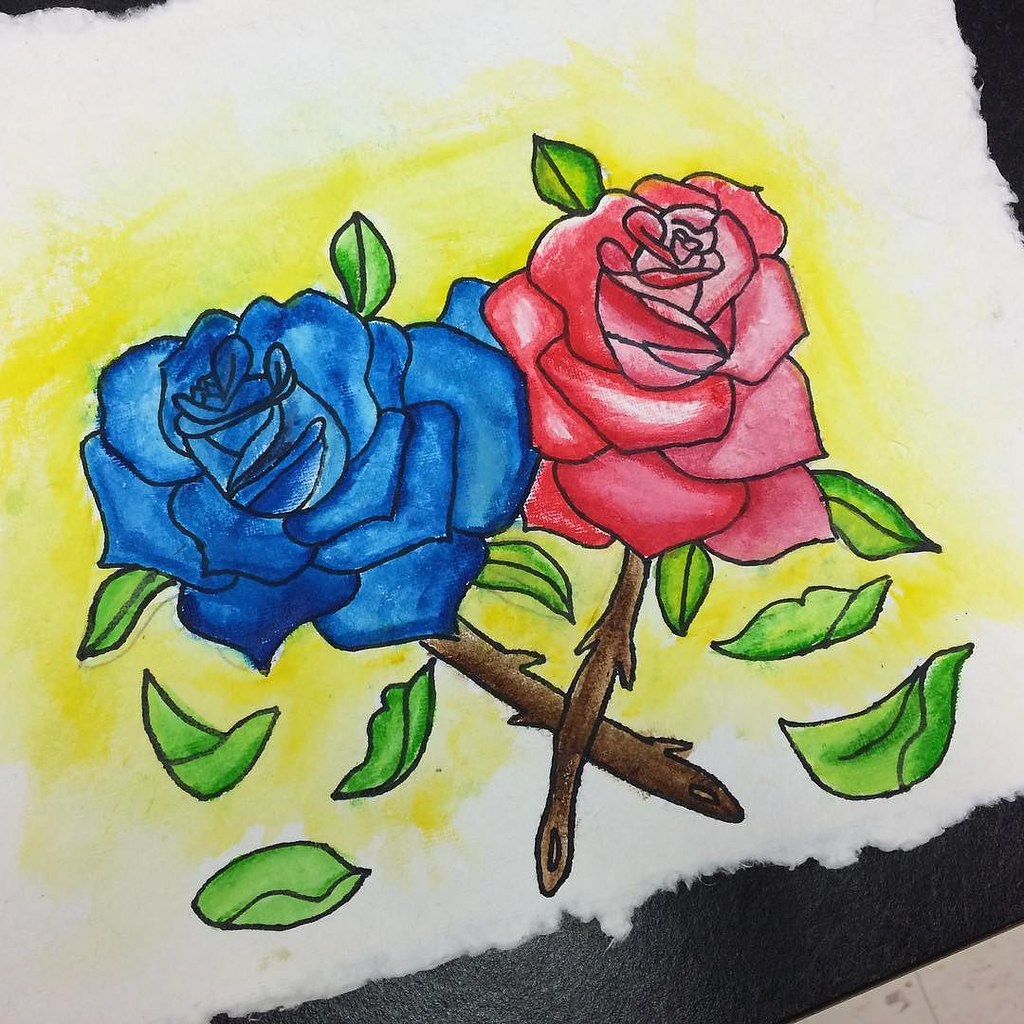This photograph captures a detailed drawing rendered on a piece of handmade paper, which is delicately frayed and fluffy along the bottom and corners. The drawing showcases two roses, their stems intertwined in an artful crisscross pattern. The stems are a deep brown, adorned with menacing thorns. The rose on the right boasts a vibrant red hue with hints of pink, while its counterpart on the left is a striking shade of blue. Several green leaves appear to be gently falling from the blossoms, adding a sense of movement to the composition. The background features a soft yellow glow, potentially suggesting either a window backdrop or sunlight illuminating the roses. This exquisite artwork is laid atop a sleek, black leather sketchbook, enhancing its presentation.